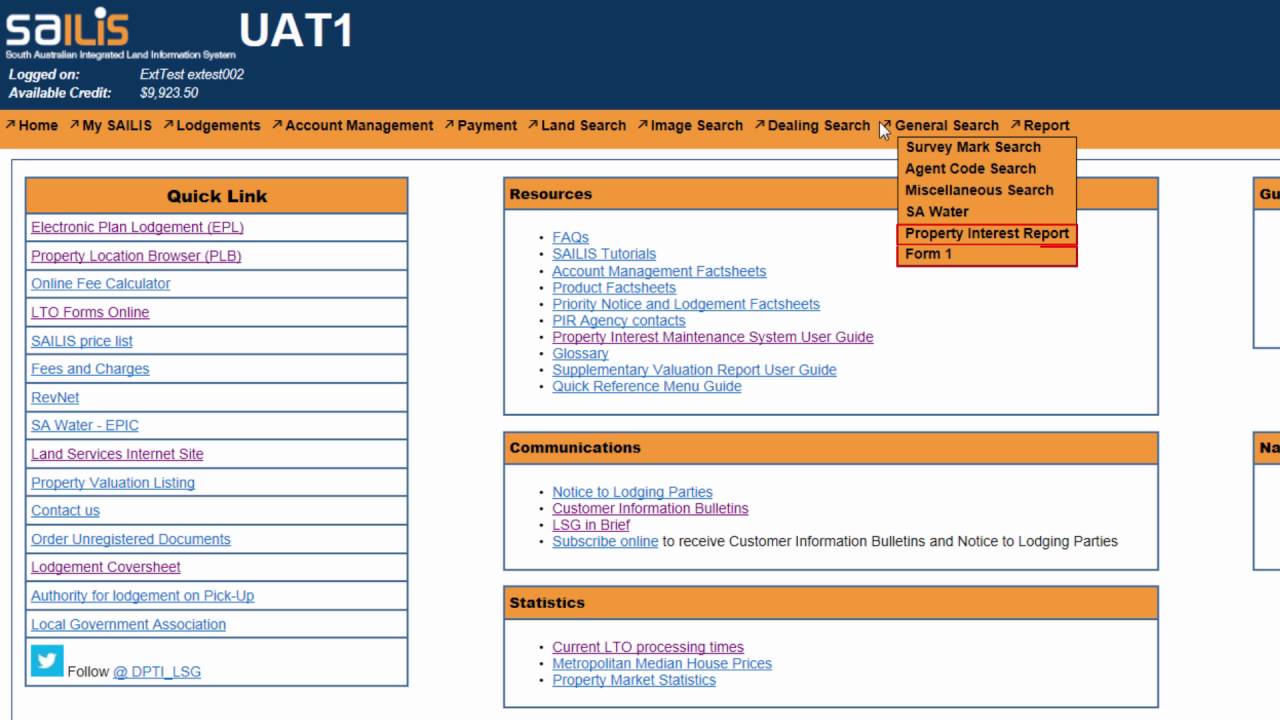This image depicts a web page from "Salis" (S-A-I-L-I-S). The logo is positioned in the upper left corner, with the "S-A" in white and the "I-L-I-S" in orange, set within a dark blue navigation bar that stretches across the top. Prominently displayed on this bar in large letters is the text "U-A-T-1."

Beneath the dark blue bar, there is an orange navigation bar featuring menu options: "Home," "My Salis," "Lodgements," "Account Management," "Payment," "Land Search," "Image Search," "Dealing Search," and "General Search." The "General Search" menu includes a dropdown box with additional options: "Survey Mark Search," "Agent Code Search," "Miscellaneous Search," "S-A-Water," "Property Interest Report," and "Form 1."

The main content area of the page is divided into four boxes, each providing different navigational options. These boxes are outlined in black. The text within the boxes is predominantly blue, with certain elements highlighted in a pink color and some text underlined. At the top of each box, the primary headings—"Resource," "Communications," and "Statistics"—are displayed in orange.